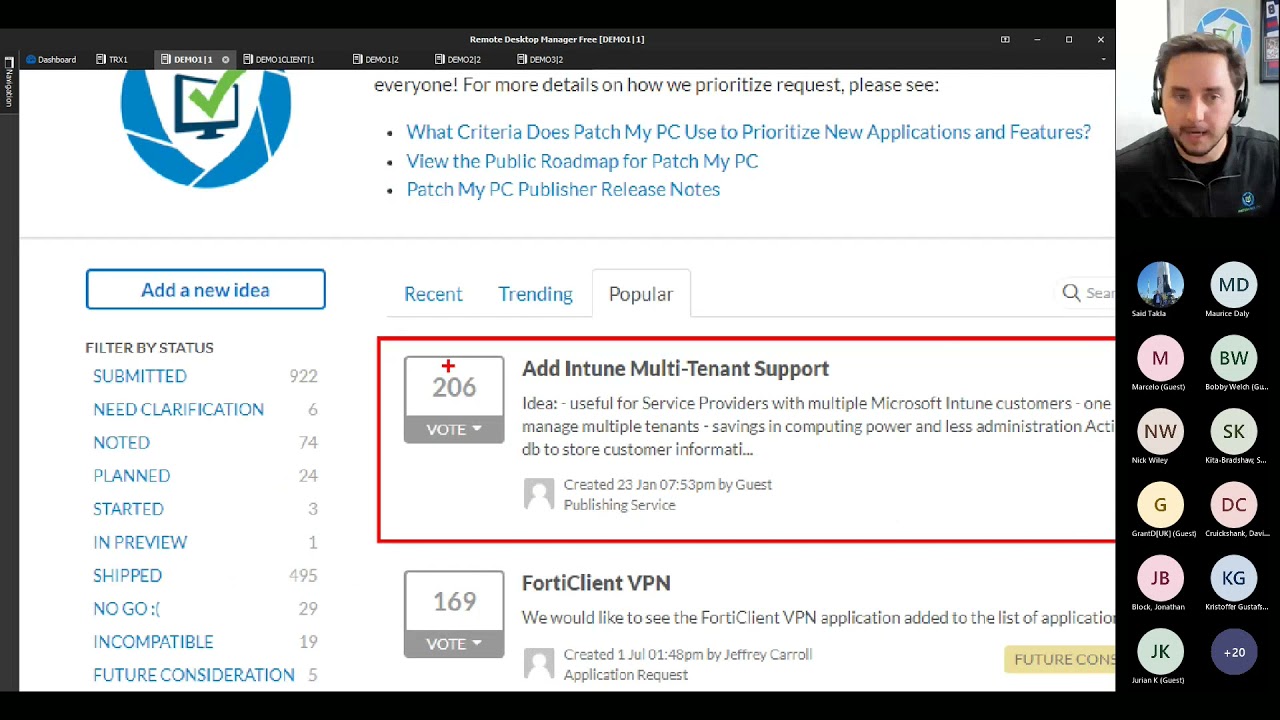The image is a screenshot of the Patch My PC website. At the top, partially cut off, is a section that reads, "For more details on how we prioritize requests, please see..." followed by the heading "What criteria does Match My PC use to prioritize new applications and features?" Below this, it guides users to view the "public roadmap for Patch My PC" and the "Patch My PC Publisher release notes."

Prominently featured on the right side of the image is a picture of a man wearing a headset. He has a mustache, a slight beard, and brown hair, and appears to be in the middle of a conversation. The presence of colored circles with initials suggests that he is connected to other participants in a virtual meeting or webinar.

On the lower part of the website, there's a section showing user-generated requests with vote counts. The highest-voted item is "Add Intune multi-tenant support" with 206 votes, followed by "Client VPN" which has received 169 votes. 

Additionally, to the left of these requests, there is a sidebar with options to "Add a new idea" and "Filter by status." The filter options include various stages of request processing: "Submitted," "Need clarification," "Noted," "Planned," "Started," "In Preview," "Shipped," "No Go," "Incompatible," and "Future consideration."

This detailed depiction illustrates the functionalities and ongoing interactive activities on the Patch My PC platform.